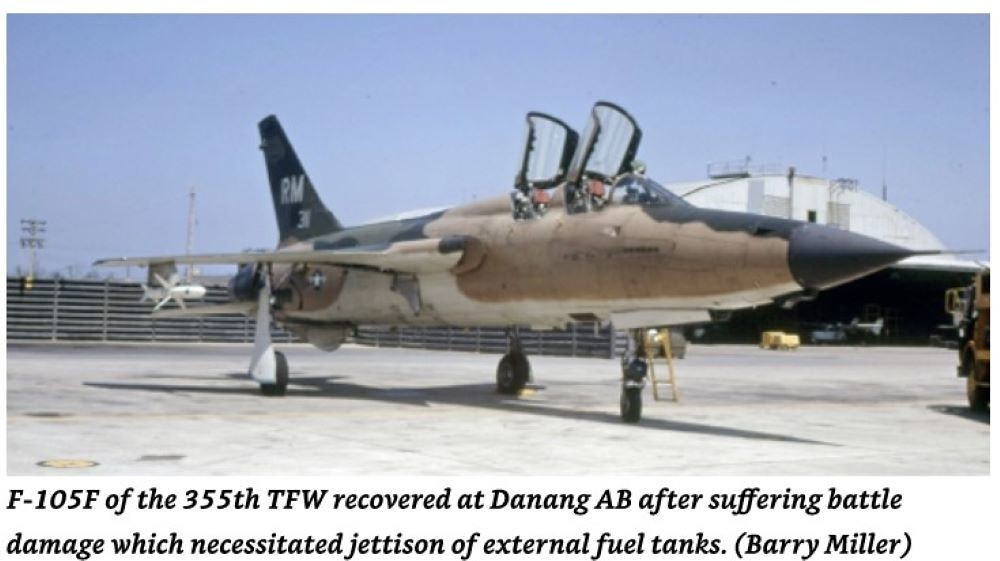This horizontally aligned rectangular photograph captures a military fighter jet, an F-105F of the 355th Tactical Fighter Wing, prominently positioned at the center of the image. The aircraft, which features a distinct color scheme with a dark brown or gray front tip, light brown sides and wings, and a dark gray tail, is parked on a concrete runway. Its canopy is open, indicating that it is a two-seater with elevated windows for both the pilot and the navigator. The setting appears to be outdoors in the middle of the day at Da Nang Air Base after the jet suffered battle damage, necessitating the jettison of external fuel tanks. In the background, the clear blue sky stretches across the top of the image, with no clouds visible. To the rear, part of a domed white and gray building is visible, along with a perimeter fence and several tall lights on poles. Directly below the image, bold black text is left-aligned, reading: "F-105F of the 355th TFW recovered at Da Nang AB after suffering battle damage, which necessitated jettison of external fuel tanks. (Barry Miller)." The various color elements in the photograph include blue, white, tan, black, gray, and yellow.